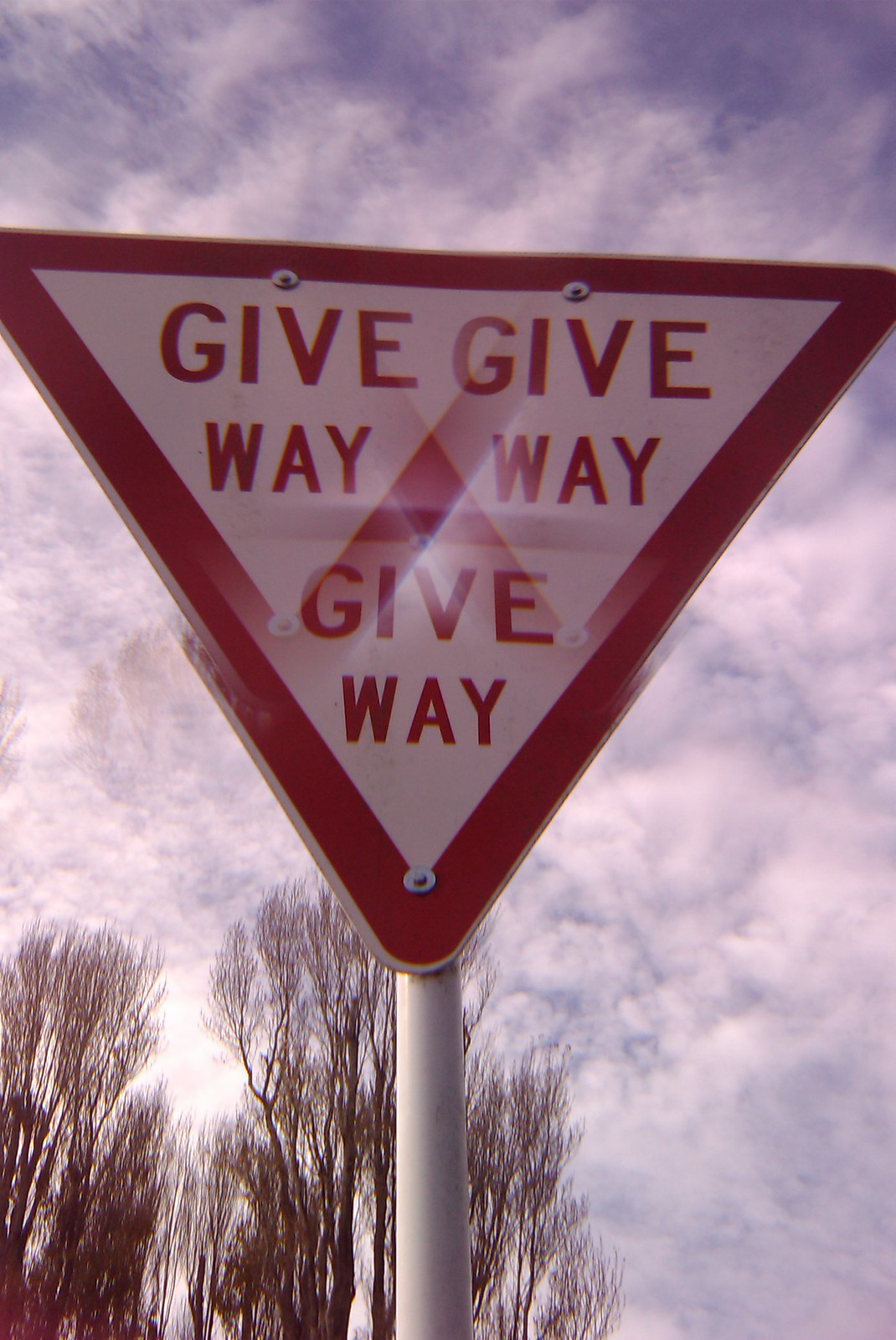The photograph captures an outdoor scene with a blue sky lightly veiled by clouds, subtly tinted with pink hues. In the lower left corner, the tops of dry, brown trees are visible. Standing prominently in the scene is a road sign mounted on a white metal pole. The sign is an upside-down triangle with a red border, signaling "Give Way." Interestingly, the sign appears to exhibit odd visual glitches, displaying the "Give Way" message three times, forming a larger triangle through the arrangement of two smaller triangles at the top and one at the bottom. Additionally, a peculiar reflection of the trees floats higher up in the sky, adding to the surreal quality of the image.